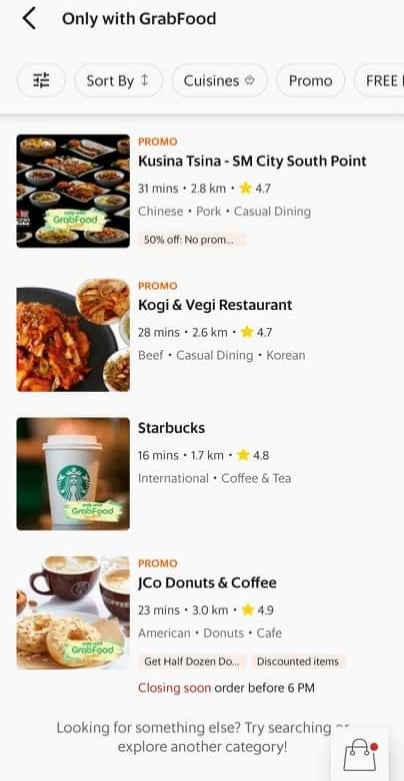This image is a screenshot taken from a cell phone, capturing a segment of a food delivery app interface. At the top of the screen, the text "only with Grab Vest" is visible, indicating a specific category or promotion. Below this header, there are filter options labeled as "Sort By," "Cuisines," "Promo," and "Free," although the last option is partially cut off.

Scrolling down, the first section highlights a promotion, prominently displaying "Fogo," accompanied by the text “Kushina Tisinin, SM Country or City South Point,” noted as being updated 31 minutes ago. The distance is listed as 38 KM.

Further down, there is a listing for "Carry and Veggie Restaurant," followed by another entry for "Starbucks." 

Continuing through the list, another promo is shown with the text "See wait…J.Co Donut and Coffee," though the full line is not captured.

At the bottom of the screen, the text encourages further exploration with "Looking for something else? Try searching," and a final prompt to "Explore another category."

This detailed screenshot provides insight into the user interface and available options within the food delivery app at a specific moment.